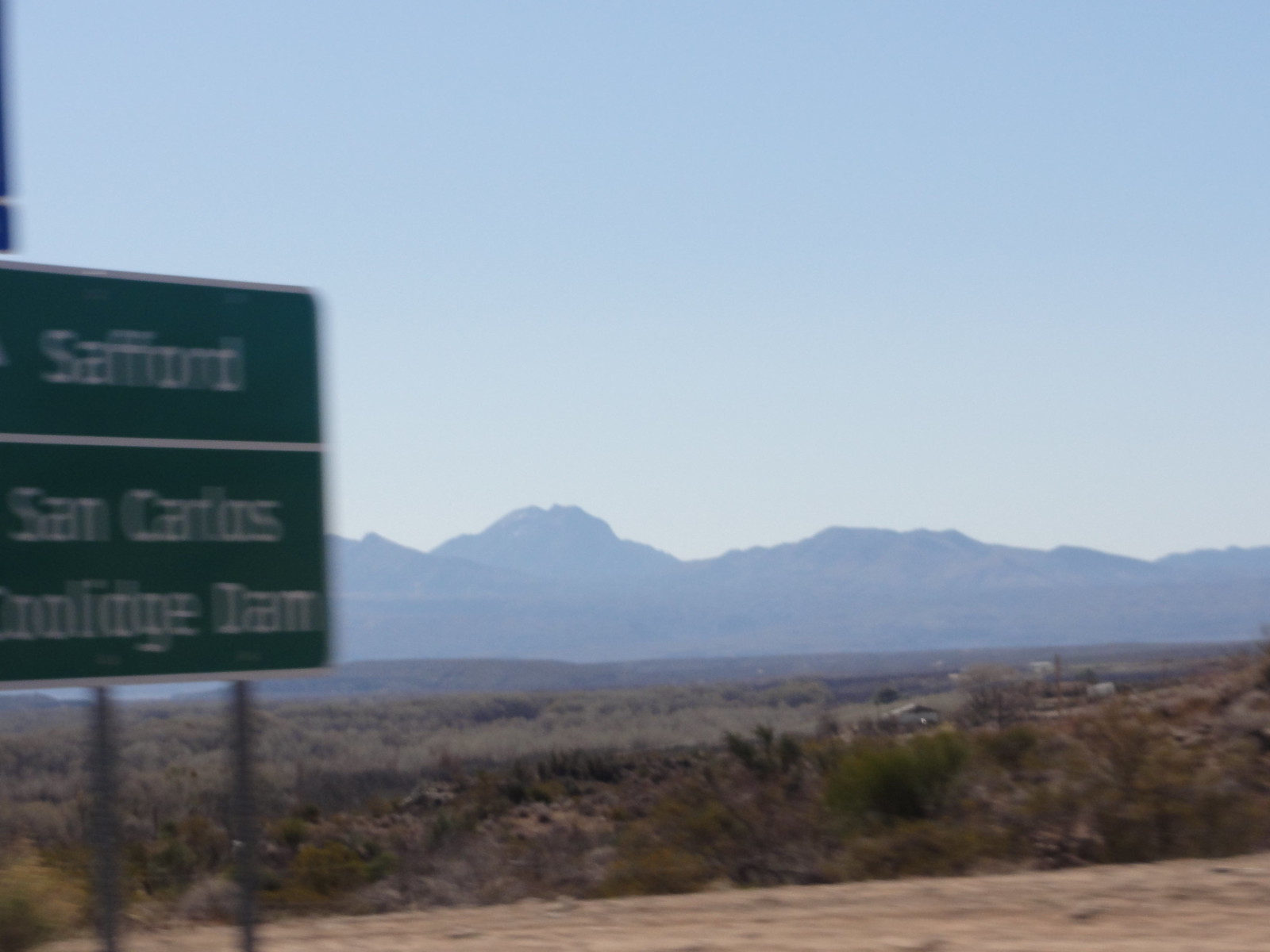This photo, taken during the daytime, captures a vast desert landscape. The foreground features a ground scattered with small hills, desert weeds, and bushes, giving a rugged texture to the scene. In the distance, a majestic mountain range stretches across the horizon under a sky that appears whitish in color. To the left side of the image, partially visible, is a green road sign with white lettering, suggesting locations like Safford and San Carlos, though the text is somewhat blurred. This blur, along with the presence of the road sign, indicates the photo was likely taken from inside a moving vehicle.